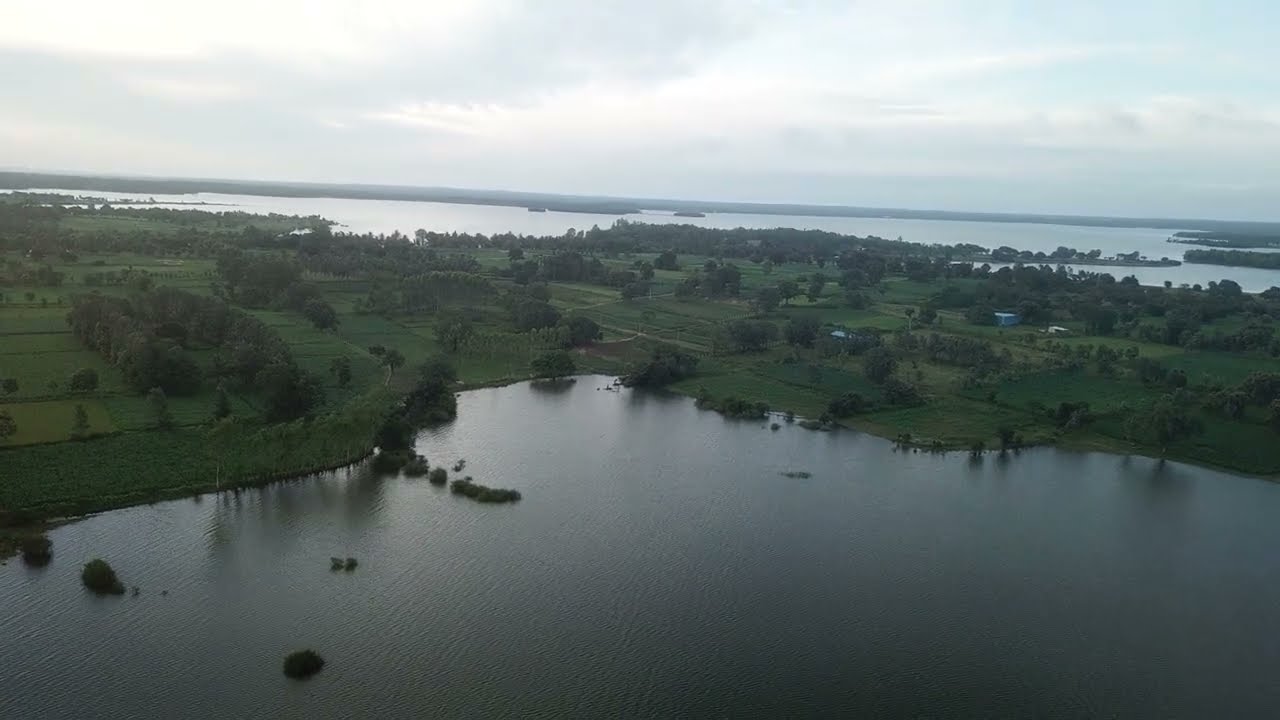This color photograph, taken from a drone, captures a serene coastal landscape in the middle of the day. At the bottom of the image, a curvy pond or estuary with bluish-gray water winds through the scenery, flanked by grassy areas, shrubs, and small trees. The central portion of the image showcases an expansive stretch of farmland, featuring plots of land interspersed with trees and a few scattered buildings, possibly houses. Farther in the distance, another body of water can be seen, extending towards the horizon. The horizon line itself is a thin strip of land or possibly more water, shrouded in ambiguity. Above this, the sky dominates the upper portion of the image, filled with streaky gray and white clouds that contrast with patches of blue. The image encapsulates the beauty of nature's open fields and waterways, emphasizing the harmony between land and water under a partly cloudy sky.